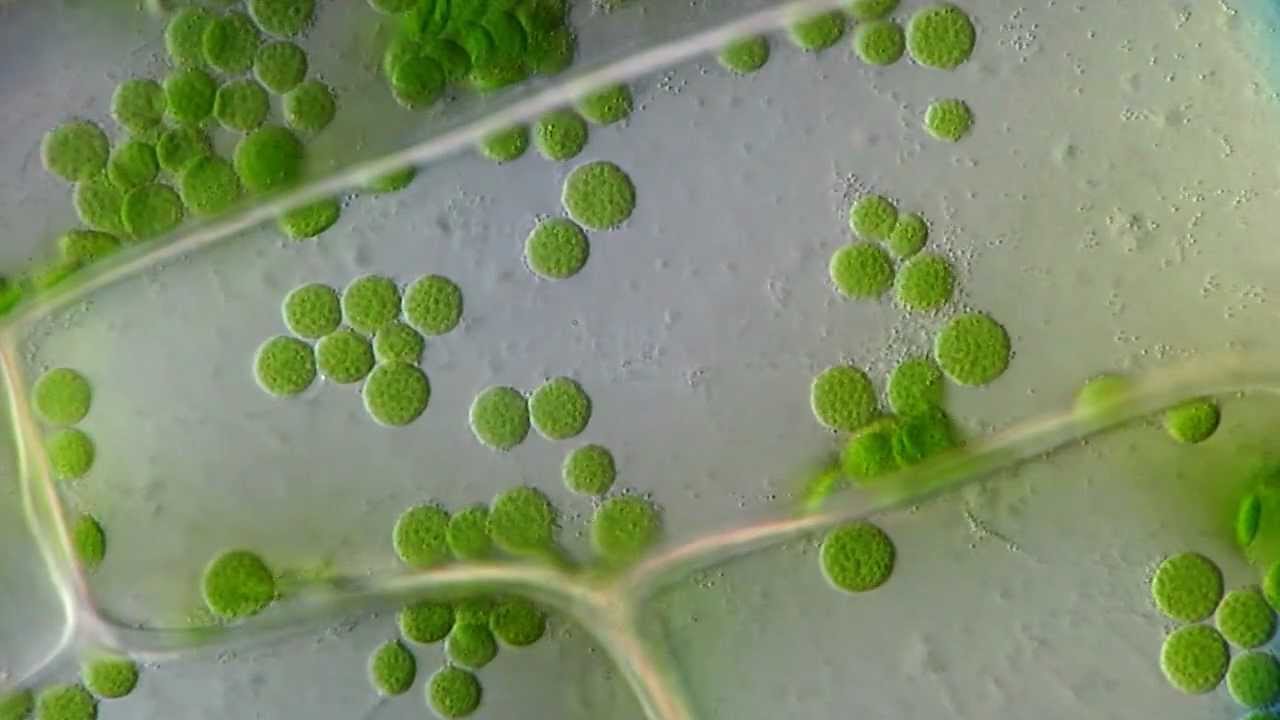The image appears to be a close-up view, possibly under a microscope, showcasing an intricate scene of bright lime green circular objects that resemble cells or bacteria. These lime green circles are scattered throughout a grayish background, with a noticeable clustering in various parts of the image, particularly in the upper left-hand corner, as well as just below a prominent, raised, and somewhat rectangular or rearview mirror-shaped structure. This structure seems to float above the circles and has a thin, clear layer that might suggest the presence of a liquid, confirmed by visible bubbles and blurbs. Within this rectangular shape, the green circles are more sparsely distributed compared to the areas outside and beneath it. The background also features a subtle, pointed 3D texture emanating from a white area, adding further complexity to the scene. Overall, the image evokes a scientific, possibly biological, microscopic context.